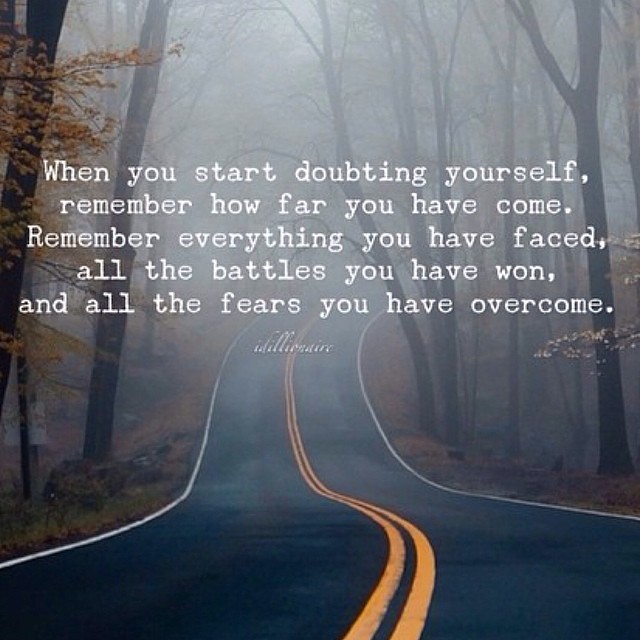In this image, there's a picturesque country road flanked by trees with a mix of bare branches and dried leaves. The road is clearly marked with two bold orange lines in the center and white lines on the edges, suggesting a well-maintained, two-way path. As the road winds through the misty and foggy forest, it slopes gently downhill before leveling out. Hovering over this serene background is an inspirational quote rendered in a clean white serif font, reminiscent of typewriter text, which starkly contrasts against the darker, earthy tones of the scene. The quote reads, "When you start doubting yourself, remember how far you have come. Remember everything you have faced, all the battles you have won, and all the fears you have overcome." Beneath these motivating words is an illegible signature in a smaller script font, adding a personal touch to the message. The overall image exudes a sense of calm and encouragement, making it an ideal candidate for social media sharing.